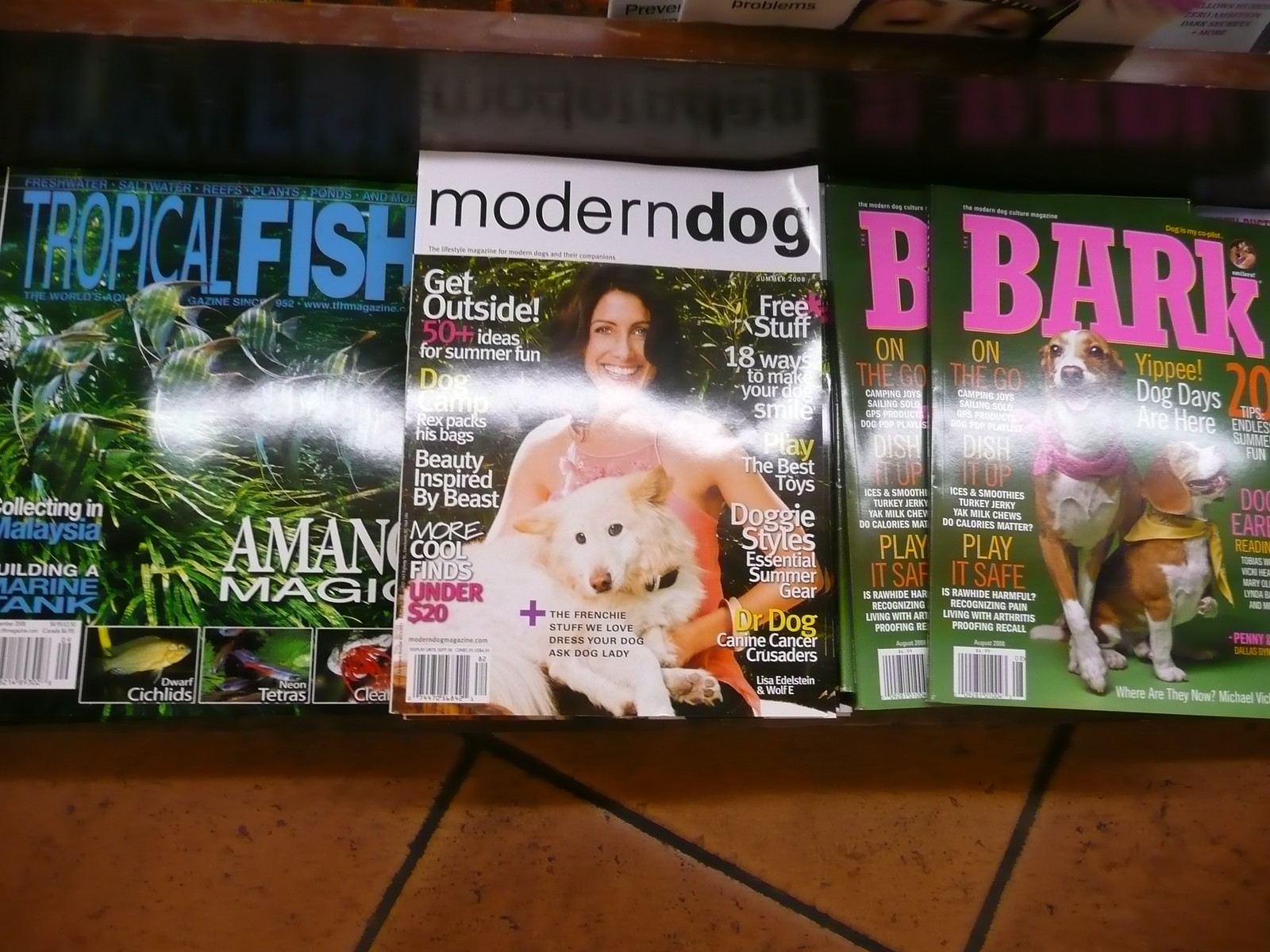In this indoor setting, a rectangular photograph captures three magazines laid out side by side on a medium brown tiled surface with dark grout lines. On the left, the cover of "Tropical Fish" features green fish illustrations and labels along the bottom, including a notable tetra fish, along with text about building a marine tank. The middle magazine, "Modern Dog," showcases a smiling dark-haired woman holding a white dog with a brown nose and black eyes, accompanied by captivating headlines such as "More Cool Finds Under $20," "Beauty Inspired by the Beast," and "50 Plus Ideas for Summer Fun." The rightmost magazine, titled "Bark" in bold pink letters, displays two dogs—one a beagle and the other a similar but taller breed—both adorned with small scarves around their necks. The scene is backed by a wooden ledge, potentially suggesting a storage area for the magazines.